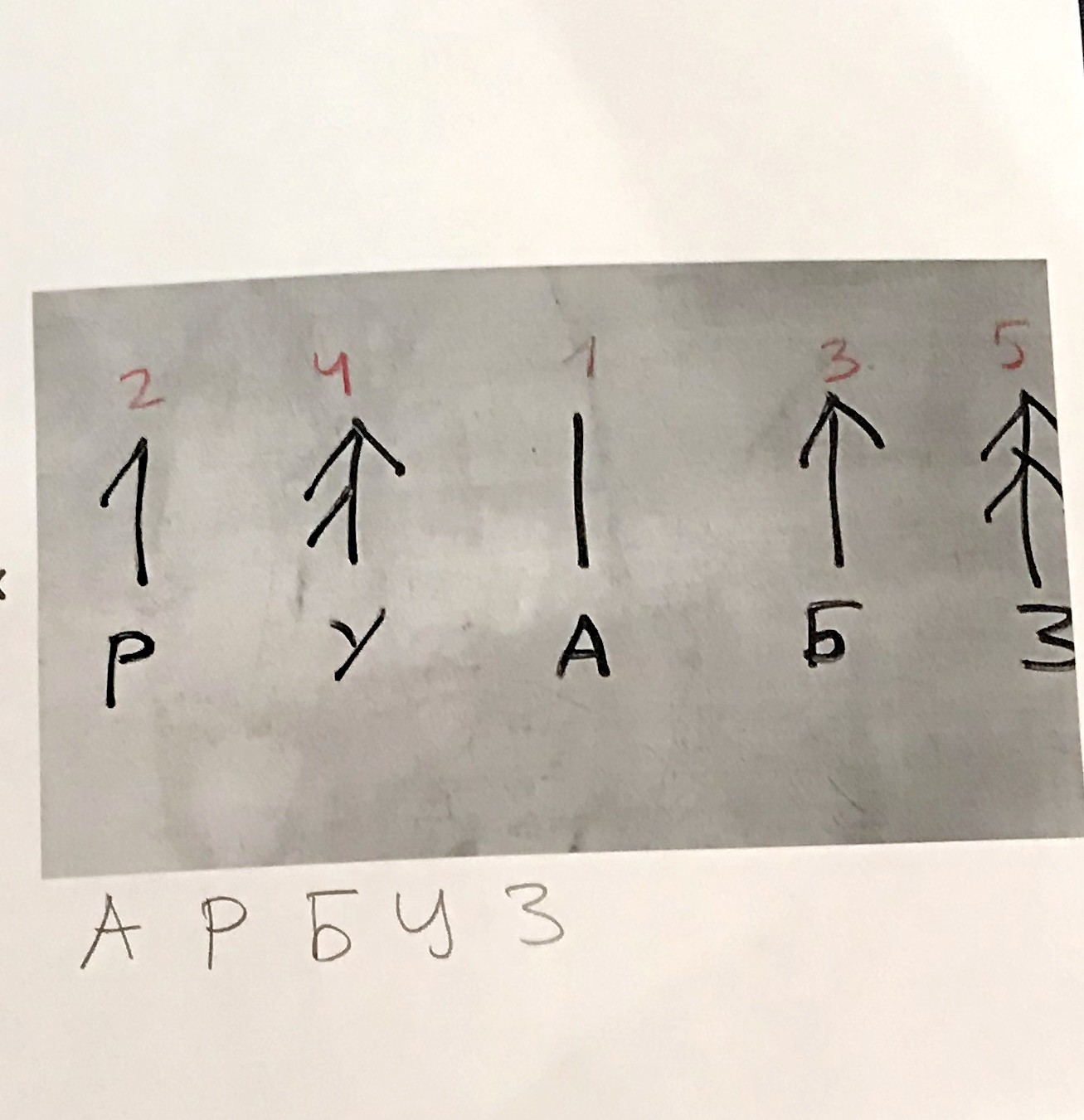This photograph captures two pieces of paper on a white background. The first piece of paper features the following sequence of characters: "A, P, B (or 5), Y, 3." Meanwhile, the second piece of paper has a slightly different texture with a whitish-gray coloring, possibly indicating it is either worn or just naturally looks that way. This piece contains three distinct rows of writing. 

In the top row, a set of red numbers reads: "2, 4 (or a similar shape), 1, 3, 5". The second row consists of various arrow-like symbols: 
- Under the "2," there is a vertical line with a single mark on the left side at the top, forming a partial arrow.
- Under the "4," there is a more standard arrow with two marks at the top and an additional mark on the left side.
- Under the "1," there is a simple vertical line.
- Under the "3," there is a classic arrow symbol.
- Under the "5," there is a double arrow with two arrowheads stacked one beneath the other.

The third row features individually corresponding characters beneath each symbol:
- Under the "2" symbol is a "P."
- Under the "4" symbol is a "Y."
- Under the "1" symbol is an "A."
- Under the "3" symbol is a character that could be a "5."
- Under the "5" symbol is a "3."